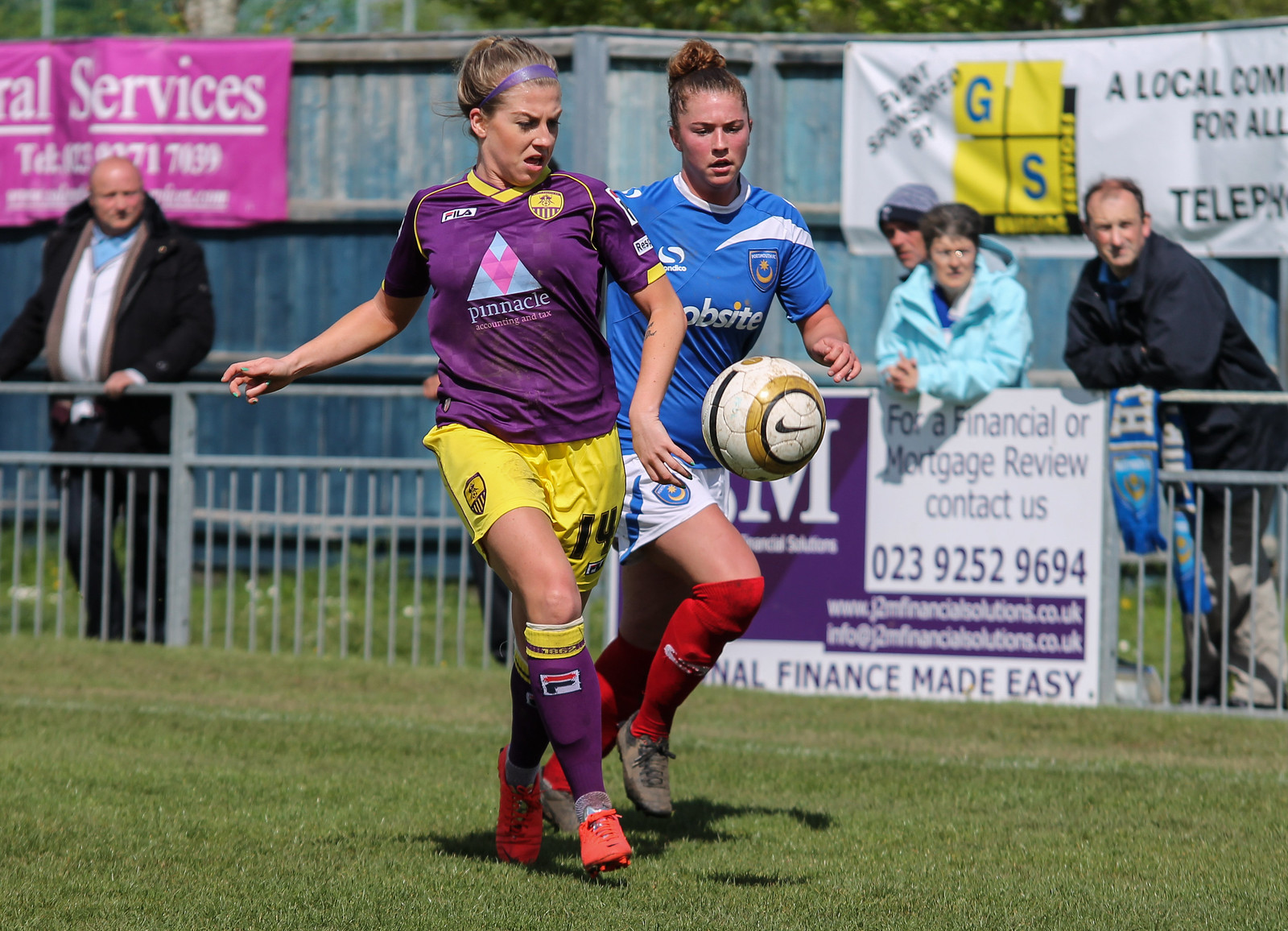This horizontally aligned rectangular picture depicts an intense soccer match between two young women, likely in their early 20s, on a lush green field marked with white sideline stripes. The action centers on the two players: the one on the left, with blonde hair tied back by a purple headband, dons a predominantly purple jersey with the word "Pinnacle" and a blue triangle, accompanied by yellow shorts and purple socks. Her red shoes are poised to kick a white Nike soccer ball adorned with gold and black stripes, her mouth open in exertion. The opponent on the right, whose brown hair is secured in a bun, is clad in a blue and white jersey that says "Jobsite," white shorts, and red socks. She races alongside, aiming to intercept the ball.

The background narrates a vivid scene with a metal fence featuring vertical poles, where spectators in coats are closely watching the game. Among them, a bald man in a black jacket stands out to the left, and three other people are on the right side. Beyond the metal fence, a blue wooden fence holds advertisement banners—one hot pink with the word "services" in white letters and another white banner with a yellow box containing the letters "G" and "S" in blue. This detailed tableau captures not only the players' dynamic movement but also the engaged audience and the vibrant promotional backdrop.